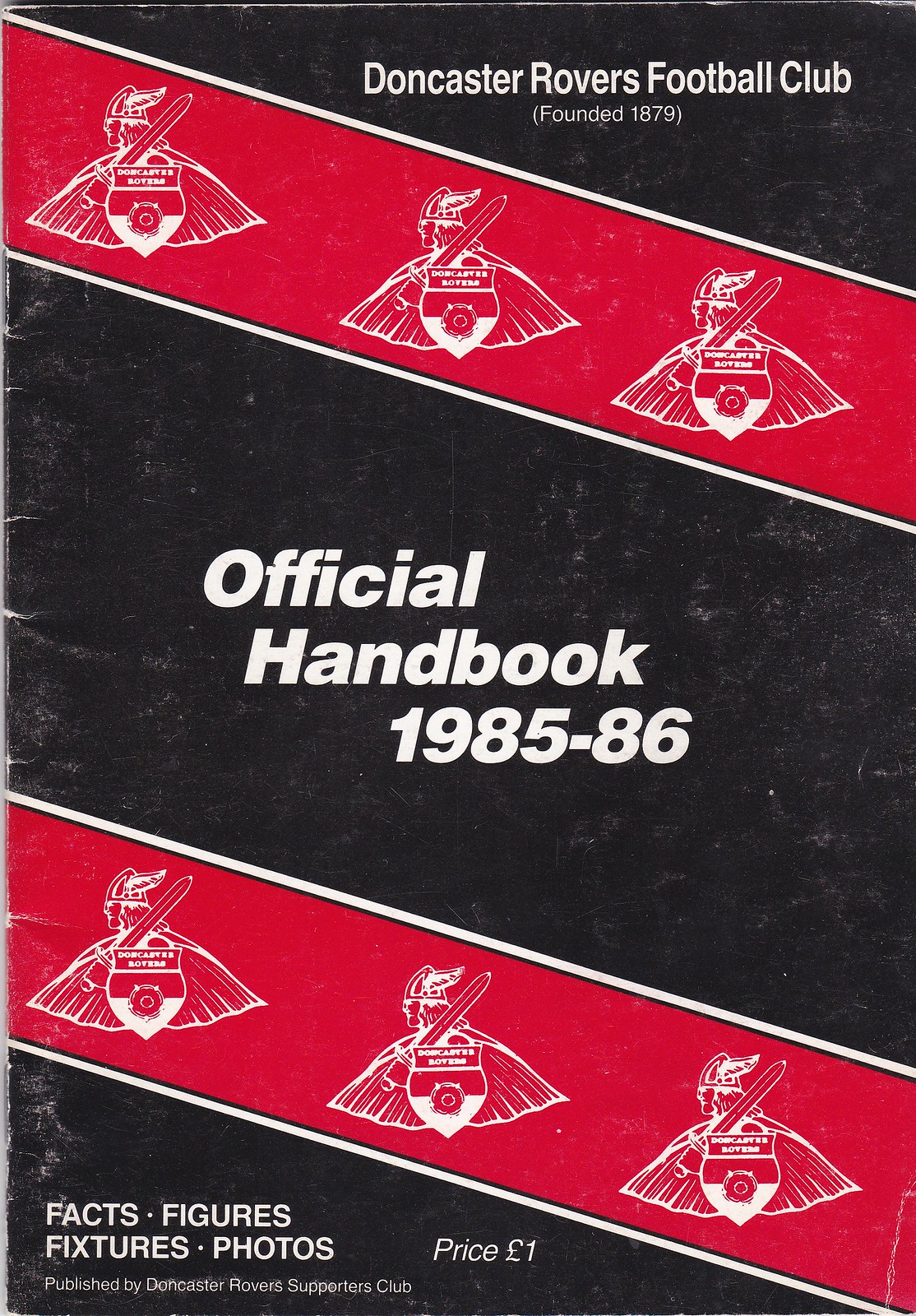The photograph depicts the cover of a handbook for Doncaster Rovers Football Club, titled "Official Handbook 1985 to 1986." The cover features a vivid design with red stripes at the top and bottom, separated by a central black strip holding the main title in white text. At the top, "Doncaster Rovers Football Club, founded 1879" is prominently displayed. The club's crest—depicting a Viking with a sword, shield, and wings—appears multiple times, with three logos positioned above and three below the central strip. The bottom left corner details additional content, stating "facts, figures, fixtures, photos" and marks the price as one pound. The booklet, bound with staples, is a fairly small publication, produced by the Doncaster Rovers Supporters Club.